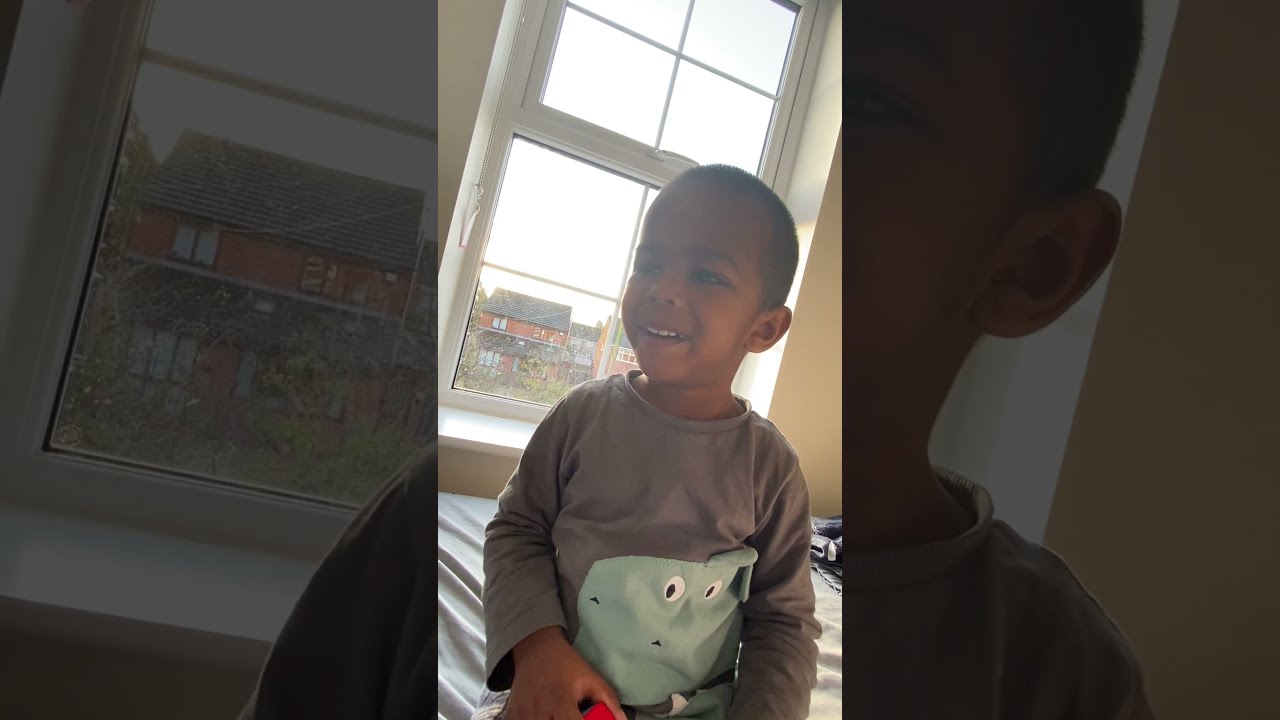The photograph is divided into three panels, with the central panel being slightly smaller than the two outer panels. The main image showcases a young boy, approximately three years old, seated on what seems to be a white bed with noticeable wrinkles on the sheets. The boy, who has dark, closely-cropped hair and brown skin, possibly of African or Indian descent, is facing forward with his head turned towards his right. His mouth is open slightly, revealing his top teeth, as though he has heard a sound. He is dressed in a long-sleeved gray shirt featuring a rectangular green dinosaur on the front.

The scene is indoors, framed by a window behind the boy that offers a glimpse outside. Through the window, a two-story red house with a slanted dark gray roof is clearly visible on the left side, along with another indistinct building. The sky outside is bright, casting natural light into the room. The window itself has white trim.

The outer panels are enlargements of the left and right sides of the central image, but they are underexposed and dark, creating a stark contrast. The left panel highlights the red house seen through the window, while the right panel magnifies the boy's face. These darkened enlargements frame the central, more vivid photograph, adding a dramatic emphasis to the boy’s curious expression.